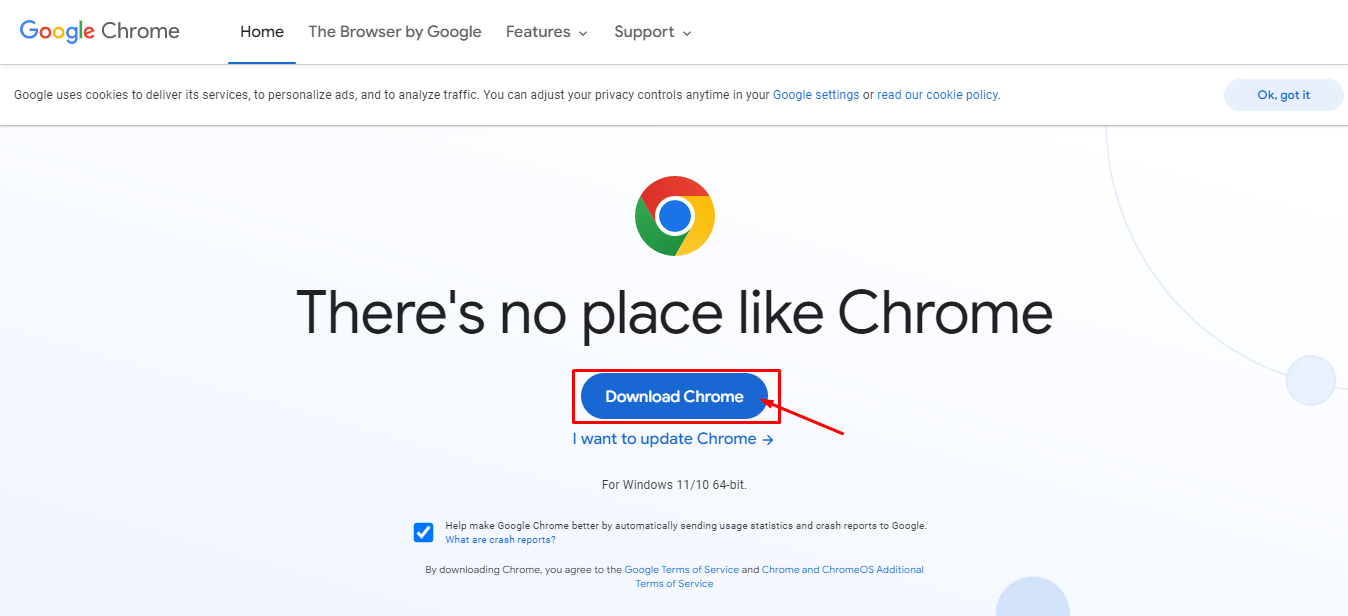This detailed image displays a Google Chrome webpage screenshot showcasing the browser’s numerous features and options. The top of the page prominently features the Google Chrome branding, with "Google Chrome" written -- each letter in "Google" decked in its respective colors: the 'G' in blue, the 'O' in red, the second 'O' in yellow, the 'g' in blue again, the 'l' in green, and the 'e' in red. "Chrome" is displayed in standard black lettering.

Below the branding, a navigation bar reads "Home," "Features" (with a down arrow), and "Support" (also with a down arrow). The "Home" tab is currently selected, highlighted by a blue underline. Beneath this is a thin black line running the page’s width, followed by another thinner black line beneath it. Nestled between these lines is a disclaimer stating, "Google uses cookies to deliver its services to personalize ads and analyze traffic. You can adjust your privacy controls anytime in your...", featuring the options "Google Settings" in black and "Read Our Cookie Policy" in blue. 

On the right-hand side, there's a light blue circular or oval icon that reads, "Okay, got it" in white. The central focus of the image is the Google Chrome icon—a circle divided into sections of green, red, and yellow with a blue center, displayed alongside a tagline, "There's no place like Chrome" in black text. Directly below this text is a dark blue oval button labeled "Download Chrome" in white, encased in a red box with a red arrow pointing to it from the right.

Further beneath the red box, a clickable link reads, "I want to update Chrome," with a right-pointing blue arrow. Additional detailed instructions state, "for Windows 11/10, 64-bit" in black. A checkbox, marked with a blue box and white checkmark, sits next to the statement, "Help make Google Chrome better by automatically sending usage statistics and crash reports to Google," in black lettering. Below this, a blue link asks, "What are crash reports?"

Concluding the web page, there's an agreement notice in black that reads, "By downloading Chrome, you agree to the," with "Google Terms of Service" and "Chrome and Chrome OS Additional Terms of Service" in blue. The text sits on an extremely light blue background. Decorative elements include a half-circle design at the upper right and another near the bottom-center-right, bordering closer to the text.

Overall, the image captures the intricacies of the Google Chrome website, complete with navigational features, download prompts, and important disclaimers.